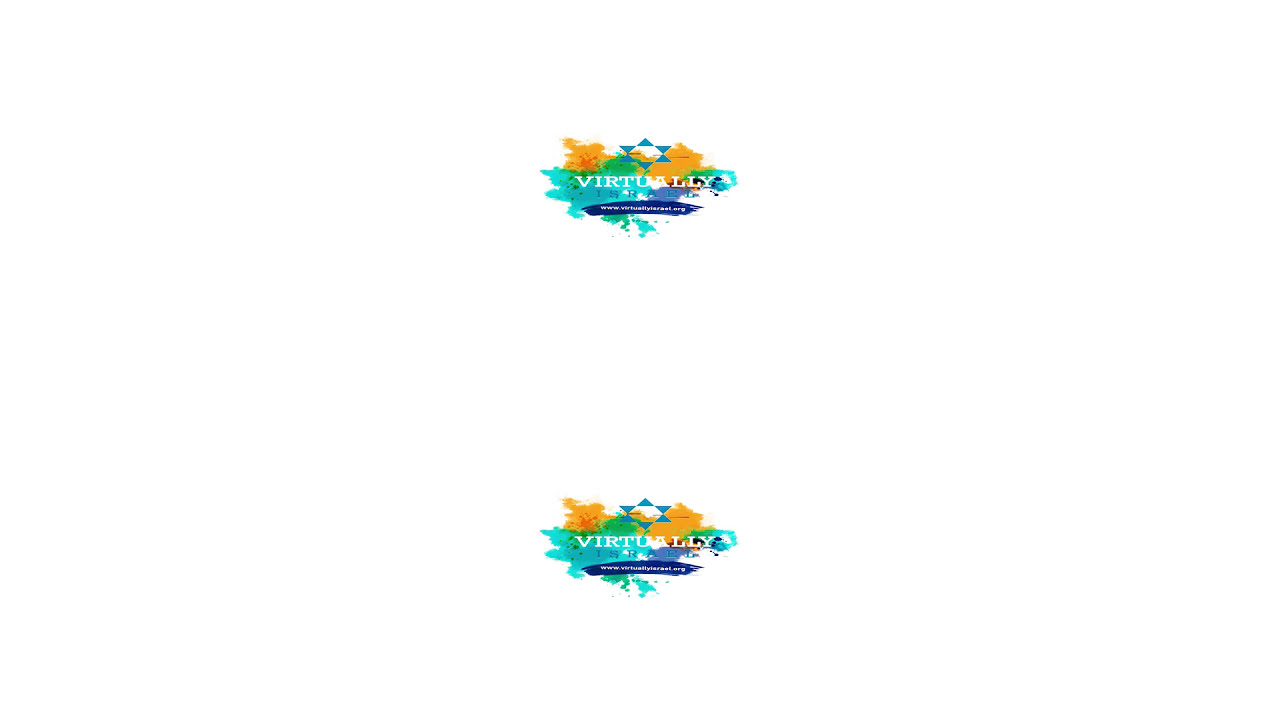This image features a duplicated logo, one positioned above the other on a white background. The logo predominantly showcases the word "VIRTUALLY" in all-capital, white serif font. Both instances of the logo include a distinctive navy blue brushstroke beneath the text. The logos are adorned with a blue star at the top, composed of six blue triangles surrounding a clear center, with a touch of yellow at the bottom. Around the star, there is a teal (aquamarine) border with gold markings, forming what appears to be an oval-shaped, jagged edge that resembles leaves. The overall design includes multi-colored accents of blue, orange, teal, and gold, contributing to a vibrant and detailed visual.